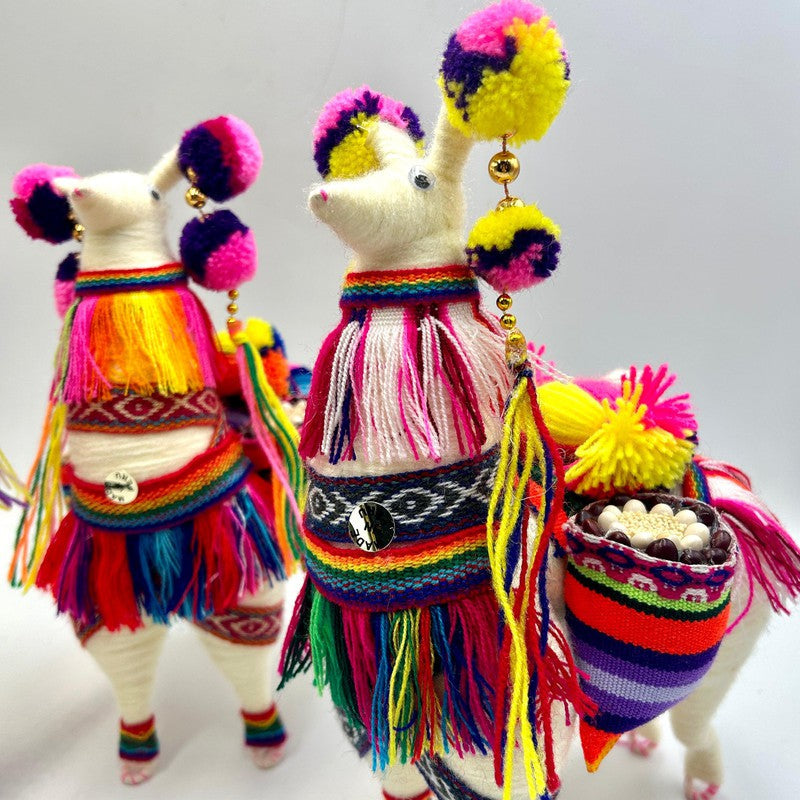The photograph depicts two handmade toy llamas crafted from yarn, featuring predominantly white bodies. They are adorned with vibrant and festive outfits, including multicolored decorations reminiscent of friendship bracelet threads that create intricate shirt-like and skirt-like patterns around their bodies. Each llama has small googly eyes and is decorated with colorful pom-poms: yellow on one and pink on the other. Gold balls and additional pom-poms dangle from their ears, enhancing their cheerful and celebratory appearance. One of the llamas also carries a rainbow-colored basket hanging from its side, adding to the playful and lively aesthetic. The background of the image transitions from a gray top to a white bottom.